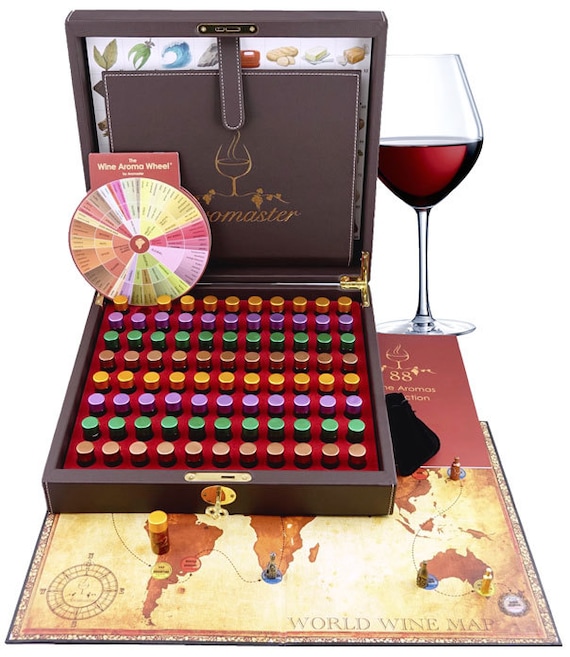The image features an unlocked, open brown box with a leather strap, resting on a white background. The box is divided into two sections but remains connected. Inside the lid of the box, there is a display with a white background illustrating various small images like fruits, leaves, an ocean wave, blocks of cheese and butter, and possibly a piece of wrapped candy. Central to this display is a simple drawing of a wine glass with red wine, accompanied by partially visible gold text that likely reads "Master."

Propped up within the upper section of the box is a multicolored "Wine Aroma Wheel" resembling a paint sample wheel, featuring colors such as white, yellow, red, pink, green, brown, tan, and orange. The lower section of the box contains rows of small flasks or cylinders arranged on a red velvet display board. The colors of these flasks are brown, green, purple, and yellow, repeating in a pattern across eight rows.

Positioned beside the open box is a tan-colored map titled "World Wine Map," depicting landmasses in an orangish-brown hue including South America, the tip of Africa, Australia, and part of East Asia. A gold key is inserted in the base of the box. Additionally, on the right side of the background, there's a clean, transparent wine glass half-filled with red wine, featuring a long stem and clearly drawn detailing.